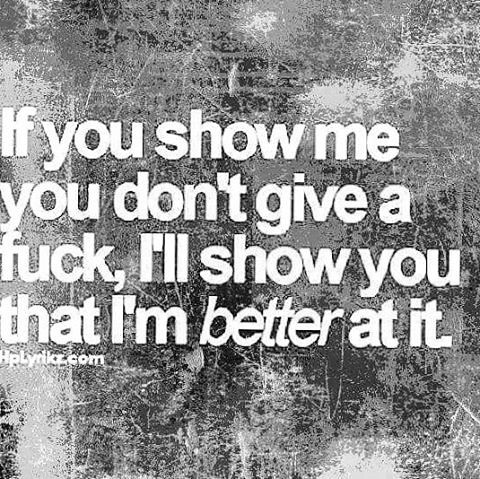The image features a black, white, and gray abstract, scratchy background reminiscent of an art piece with high contrast and visible blurs, possibly evoking a distorted vision of a forest with hints of tree branches and a dirt walkway. Dominating the center of the image is a bold white text arranged in four lines, reading: "If you show me you don't give a fuck, I'll show you that I'm better at it." The word "better" is italicized for emphasis. Beneath this quote, the text "hplyrics.com" is included, likely indicating the source or creator of the quote.